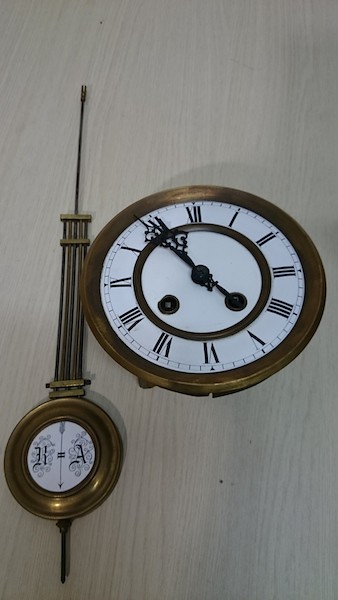This image shows a collection of intricate components that seem to belong to a grandfather clock. The parts are displayed on a surface made of whitewashed or pickled pine, which provides a rustic, bright backdrop. In the upper right-hand corner of the image, there is a large, round clock face adorned with Roman numerals and elaborate hands, indicative of a classical timepiece design. 

In the lower left-hand corner, there is a smaller, round brass piece with a white center, featuring ornate initials. The right-hand initial is a distinct "A," while the left-hand initial could be an "H" or a "K." This smaller component is pierced by an arrow, adding to its decorative complexity. It is also connected to five rods, which suggests it could be part of a pendulum mechanism, often seen beneath the face of a grandfather clock, moving rhythmically back and forth. Overall, the finely detailed elements and their arrangement evoke the intricate craftsmanship involved in creating a grand, traditional timepiece.